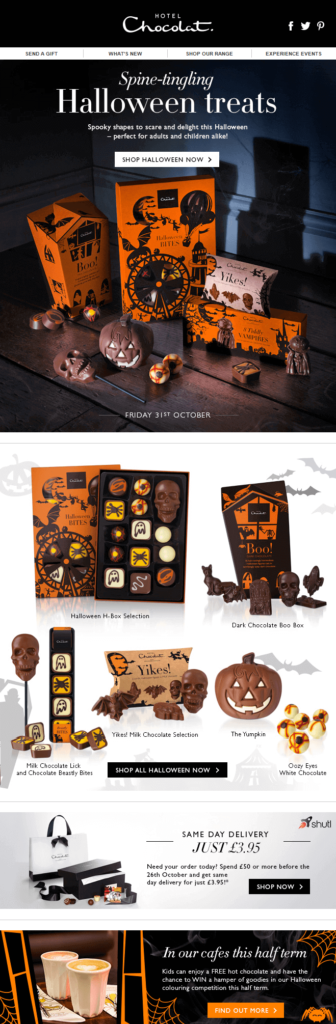**Descriptive Caption:**

The image features a black background with white text displaying the word "Hotel" and a cursive "Choc-a-lot" underneath. On the right-hand side are the Facebook, Twitter, and Pinterest logos. Below this, on a thin white strip with black text, are options to "Send a Gift," explore "What's New," and "Shop Our Range."

Dominating the image is a spooky Halloween-themed section with a predominantly purple hue, accented by orange elements and black pumpkins. At the top, in cursive, "Spine Tingling" is written, followed by regular text stating, "Halloween treats, spooky shapes to scare and delight. It's Halloween, perfect for adults and children alike." 

A black button with white text encourages viewers to "Shop Halloween Now." Below, the date "Friday, 31st October" is noted. Displayed are various Halloween-themed products, including "Too Spooky" candy sets, skull-shaped suckers, and a pumpkin-shaped chocolate treat. Same-day delivery is available for £3.95.

Further down, there are images of what appear to be lackluster cups of coffee. In white text, it mentions that "In our cafes this half term, kids can enjoy a free hot chocolate and have a chance to win a hamper of goodies in our Halloween coloring competition." Unfamiliar with "half term," a highlighted orange button invites users to "Find Out More."